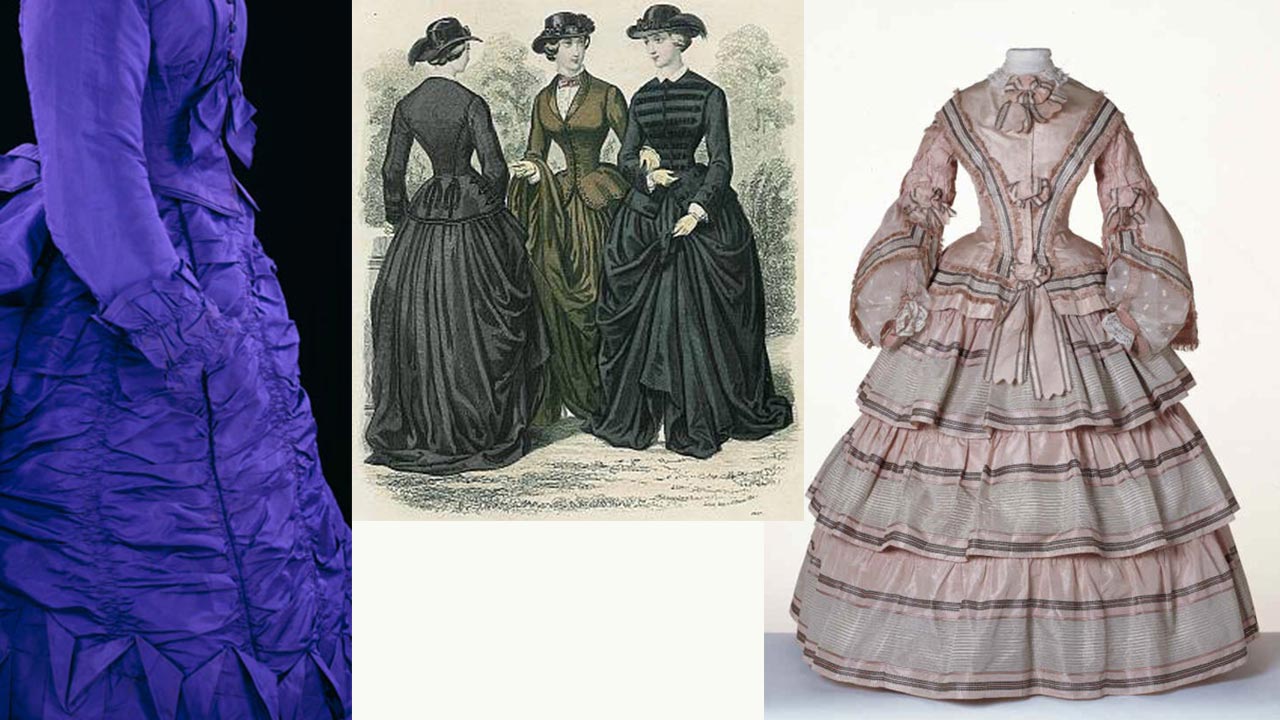This image is a detailed collage of three different representations of 18th-century Victorian dresses, positioned side by side. On the left, a vibrant, royal purple dress with a corset bodice and rippling, wrinkled fabric at the bottom is showcased. The dress is set against a pitch-black background and is shown in side profile, with a visible ribbon below the bust. In the center, there is a grayscale drawing depicting three women in similar period attire. The woman on the left, facing away from us, wears a rich black dress, while the central figure dons a dark pale green dress with a blazer-type corset and tulle-like bottom. The third woman, in another black dress, has her back turned, showing her dress tied at the back. All three women are wearing black hats. The rightmost image features a headless mannequin displaying a pink, multi-layered dress with three horizontal layers of ruffles. The dress, adorned with black frills and thin lines, widens from the hips to the floor, and includes a pink bow at the neck.